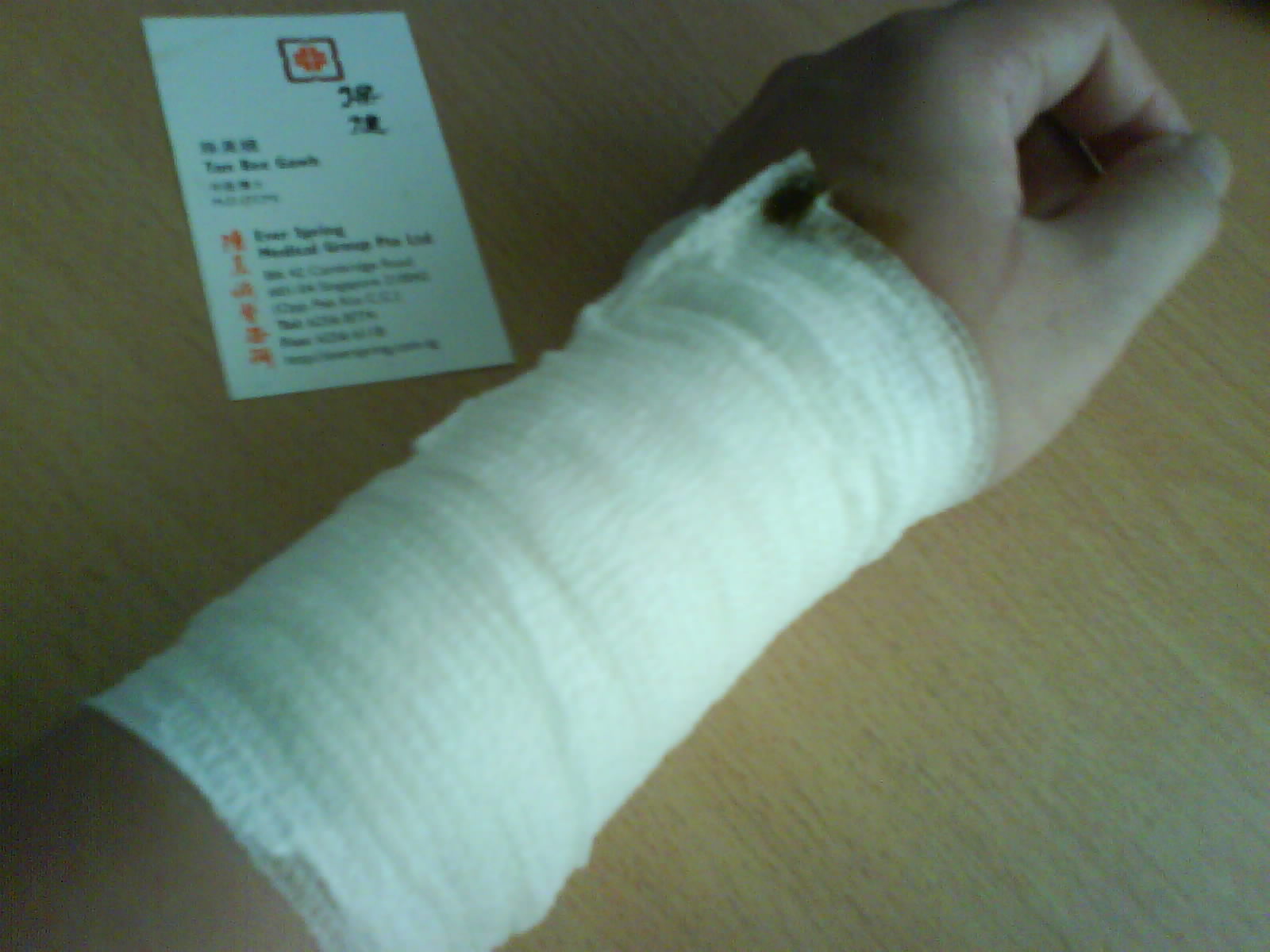This blurry color photograph shows a Caucasian person's left arm and hand, likely female, resting on a table. The arm is wrapped in a white bandage or gauze, extending from the wrist to the upper forearm, indicating an injury. There appears to be a bruise, laceration, or burn on the upper part of the hand, just above the thumb and below the pointer finger. The person’s fingers are clasped in a neutral position with the thumb on top. To the left of the arm, there is a small white rectangular card with an indistinct red logo, potentially a medical symbol, and some illegible text that might include Asian characters. Due to the poor picture quality, the details are hard to discern, but it seems to be a medical document, possibly instructions or discharge information from a medical facility.